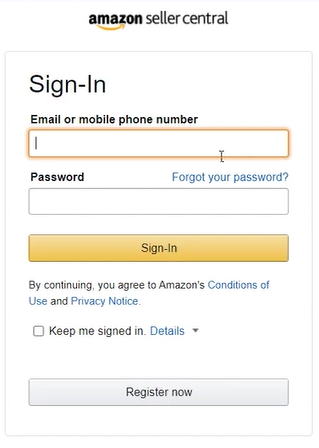Here is the cleaned-up and detailed caption:

---

This image is a screenshot from the Amazon Seller Central login page, potentially from a mobile view given the compact layout. Prominently centered at the top is the Amazon logo, featuring the word "Amazon" with the signature yellow smiley arrow underneath it. To the right, it reads "Seller Central."

Below the logo, there's a rectangular section with a light gray outline and a white background. At the top left of this section, in bold black text, it says "Sign-In," with distinct capitalization for "S" and "I," and a dash between the words.

The first input field is for the user's email or mobile phone number, marked by a bold label that reads "Email or mobile phone number." The input box is highlighted with an orange outline and a cursor inside it.

Below this, there is a second input field for the user's password, similarly marked with a bold label that reads "Password." To the right of the password field, there is a clickable text link saying "Forgot your password?" to help users who need to recover their credentials.

Beneath the password field, there's a yellow button with a gradient, labeled "Sign-In" in the center.

Further down, there is a small text block stating, "By continuing, you agree to Amazon's Conditions of Use and Privacy Notice." The text is primarily black, except for the "Conditions of Use" and "Privacy Notice" links, which are blue and clickable.

Below this text, there is a check box option labeled "Keep me signed in," followed by a blue text "Details" with a downward-facing triangle indicating additional information.

At the very bottom of the section, there is an outlined button with a gradient background, centrally labeled "Register Now" in black text, prompting new users to create an account.